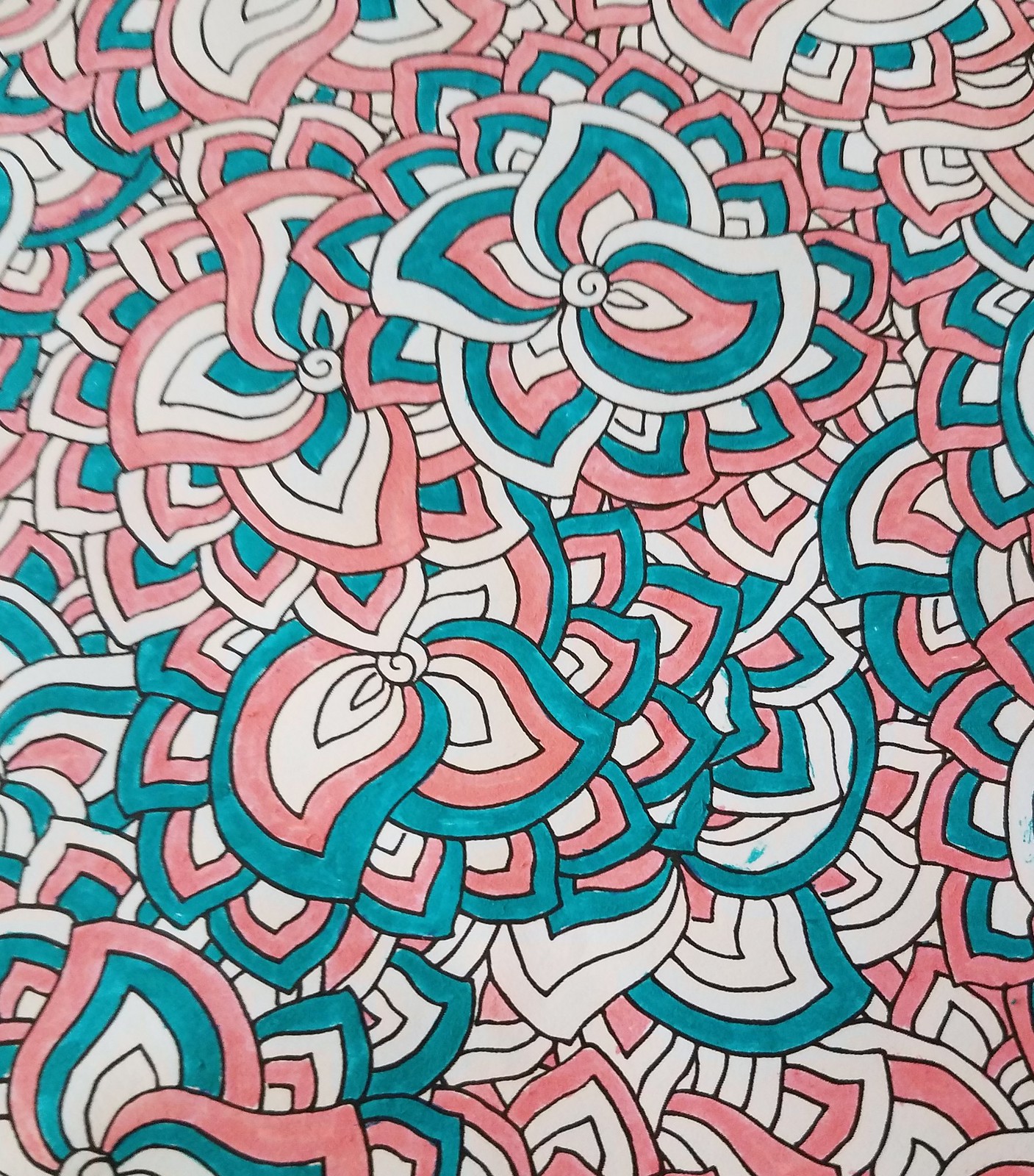This image is a photograph of a drawing on a coloring book page, characterized by an intricate pattern of four-petal flowers resembling lotuses. The flowers repeat and overlap throughout the entire page, creating a visually complex and aesthetically pleasing design. The petals are arranged in concentric circles, with the innermost layer being very light, transitioning to pastel pink, followed by turquoise, and then surrounded by another light-colored layer. The design is partially colored in with soft greens, pastel pinks, and some turquoise, with visible smudges, mostly green, suggesting the use of markers. The repeating patterns span the entire sheet, making it difficult to ascertain whether this could be wallpaper, a greeting card, or even a tablecloth. The swirly geometric shapes and harmonious color palette contribute to the image's captivating and pleasant appearance.